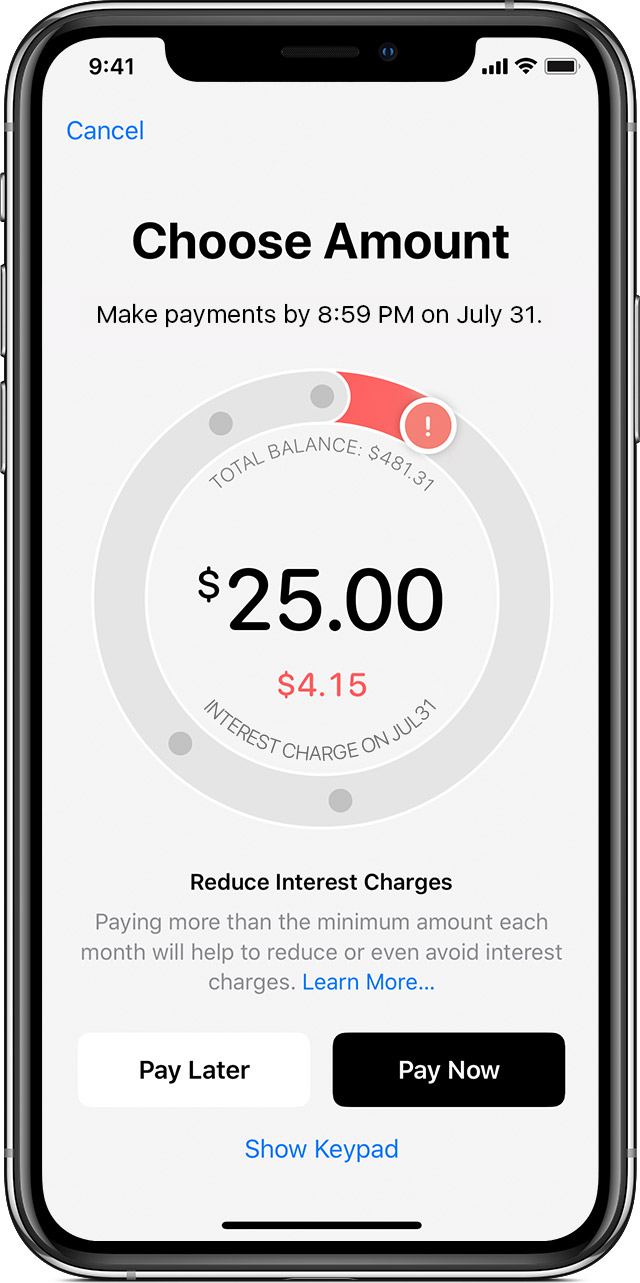This image depicts a cell phone screen displaying a payment interface. At the top, the phone shows a full battery icon and a strong connection with four bars. The time is displayed in the top left corner as 9:41. Directly beneath the time is a blue "Cancel" button.

In the middle of the screen, the interface reads "Choose Amount" in bold text. Below this, a smaller font states, "Make payments by 8:59 PM on July 31st."

Central to the image is a circle graphic that primarily appears light gray. Within this circle, text indicates that the total balance is $481.31. A small red segment at the top of the circle symbolizes a critical component, which is further highlighted by a peach-colored overlay with a white exclamation point inside it. Within this segment, it states "$25" in large black lettering, referring to the minimum payment due by July 31st, with "Interest charge on July 31st" written in red below it. 

Around the circumference of the circle, there are two pairs of gray dots—one near the middle and another pair at the top. Accompanying text advises, "Reduce interest charges: Paying more than the minimum amount each month will help to reduce or even avoid interest charges. Learn more." Below this advisory, there are options for payments: "Payments" in blue, "Pay Later," and "Pay Now" in black. Additionally, there is a blue "Show Keypad" option at the bottom.

The interface combines critical payment details, graphical representations, and intuitive options to guide the user through the payment process.